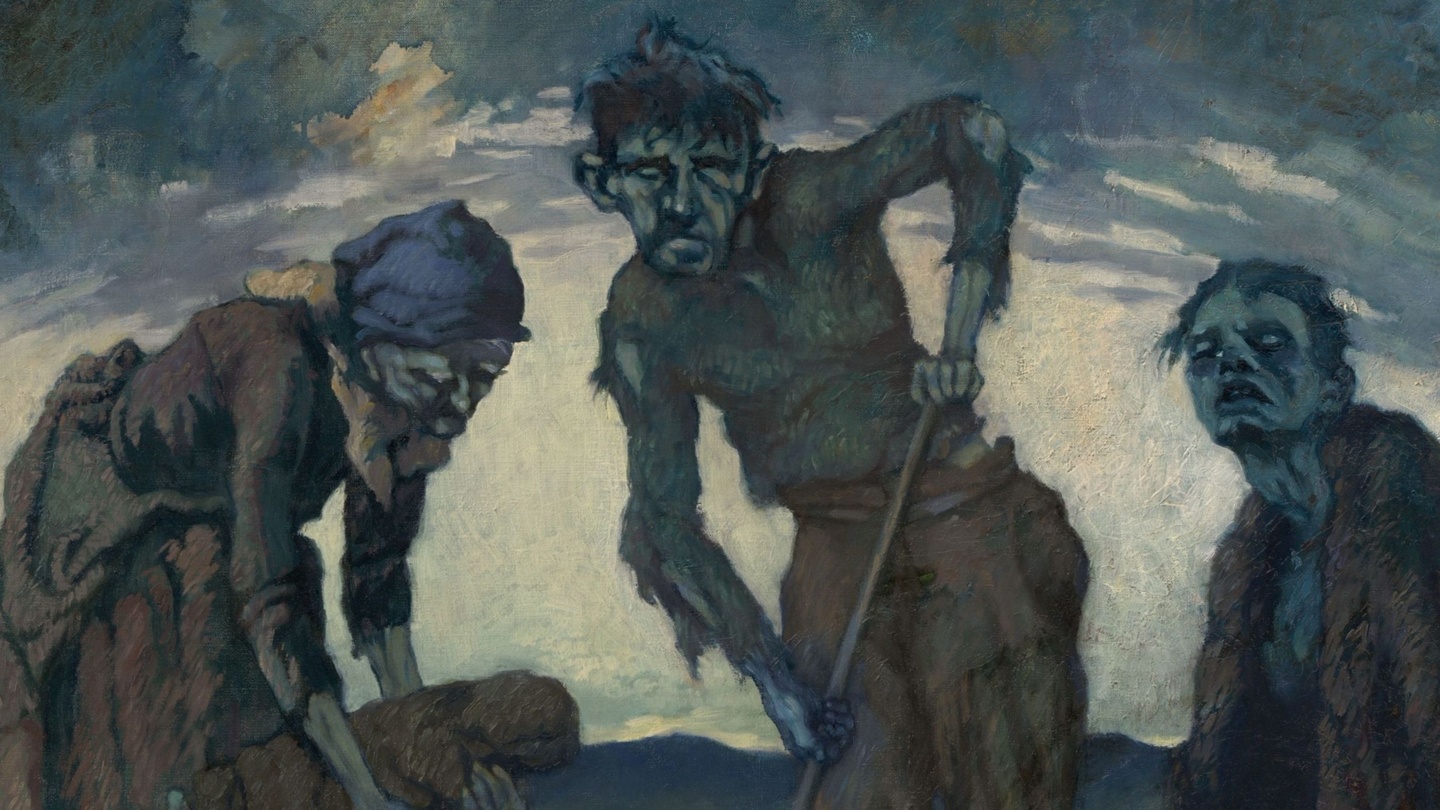The image is a dark and eerie painting set outdoors, capturing a somber and melancholic scene. The central figure is a woman wearing a long dress and a blue scarf over her head, who appears to be holding and burying a dog. Beside her stands a frail man with a torn, long-sleeve shirt and brown pants. His face is sunken, with messy black hair, and he looks sick and sad as he clutches a shovel in his hand. Another figure, a man in a brown fur coat, kneels on the ground, looking distressed with hollowed white eyes and messy hair. All three appear ghostly and destitute, dressed in ragged clothes. The overall atmosphere is very dark, dreary, and almost surreal, with the figures resembling zombies bent over their grim task, painted against a stark, contrasting black and white background.